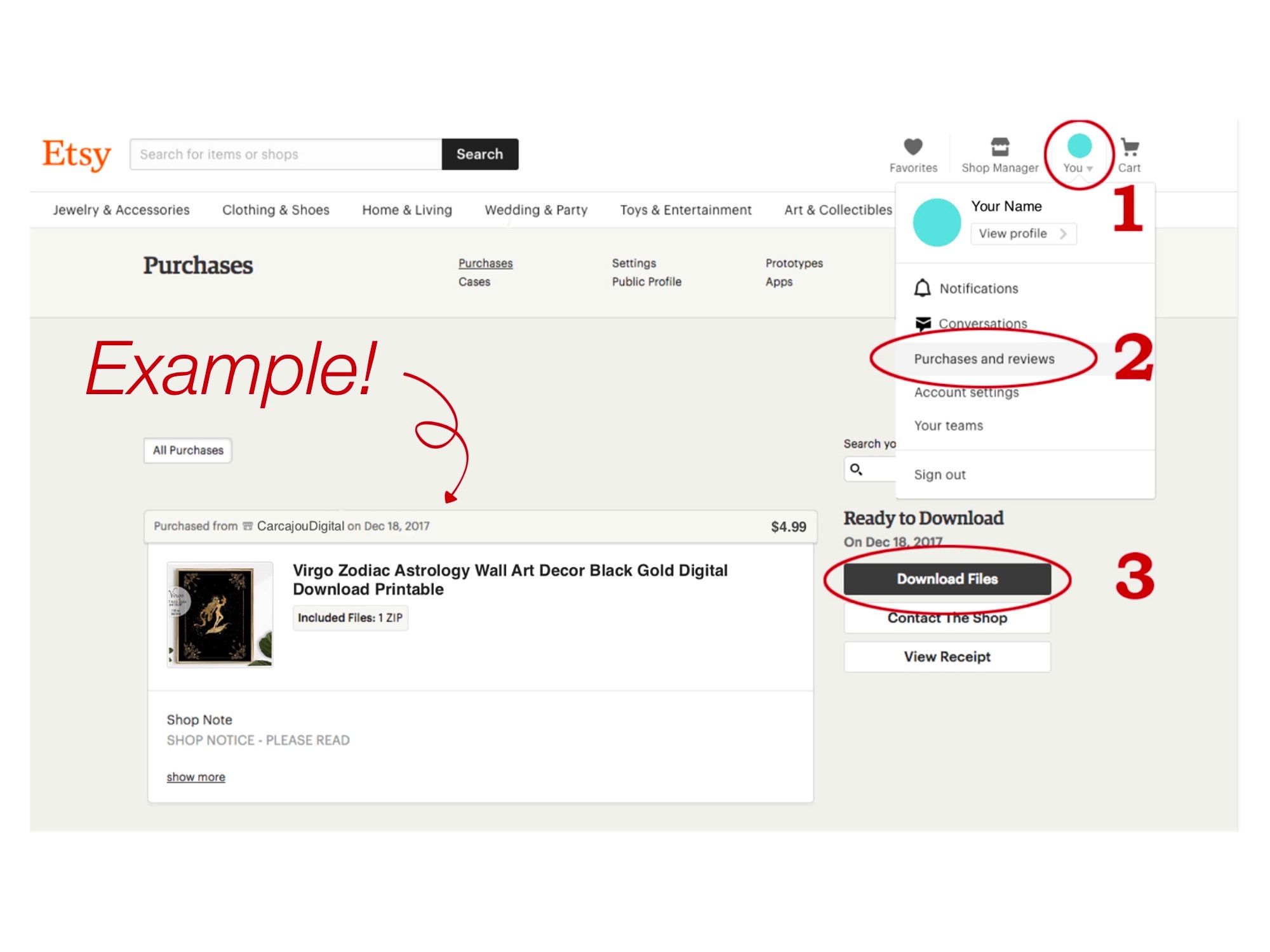**Detailed How-To Guide Screenshot Description: Etsy Page Breakdown**

The image is a comprehensive screenshot of an Etsy page, organized as a detailed how-to guide with various sections meticulously circled and labeled.

1. **Header Section:**
   - **Top Left:** The upper left corner features the word 'Etsy' prominently displayed in orange. Adjacent to it is a search bar that reads "Search for items or shops," accompanied by a black button utilized to start the search.
   
2. **User Interface Elements (Top Right):**
   - **Favorites:** Indicated by a gray heart icon labeled "Favorites."
   - **Shop Manager:** Represented by a gray storefront image icon.
   - **User Profile:** Marked with a blue circle that has "You" written on it.
   - **Cart:** Displayed as a gray cart icon.

3. **Navigation Menu:**
   - The top navigation bar includes diverse categories: Jewelry & Accessories, Clothing & Shoes, Home & Living, Wedding & Party, Toys & Entertainment, Art & Collectibles.

4. **User Dropdown Menu:**
   - Positioned below the blue "You" icon, circled in red. When expanded, it shows items such as 'Your Name', 'View Profile', highlighted by a big red number '1', indicating a notification.
   - Below this, additional options are listed including Notifications, Conversations, Purchases, and Reviews, with the label next to Notifications circled and a red number '2' signifying unread items.
   - Further down, options like Account Settings, Your Team, and Sign Out are available.

5. **Main Page Content:**
   - The main focus features a highlighted previous purchase titled "Virgo Zodiac Astrology Wall Art Decor Black Cool Digital Download Printable." This item is marked with red text that says "example."
   - A swirly arrow points towards this item, emphasizing it, and a red circle with the black download button "Download Files" is shown. A red number '3' is also placed beside this button, indicating its importance or step order in the guide.

In summary, the image meticulously shows various functional elements of an Etsy page, labeled and highlighted to serve as a comprehensive instructional guide for navigating and operating the Etsy interface.